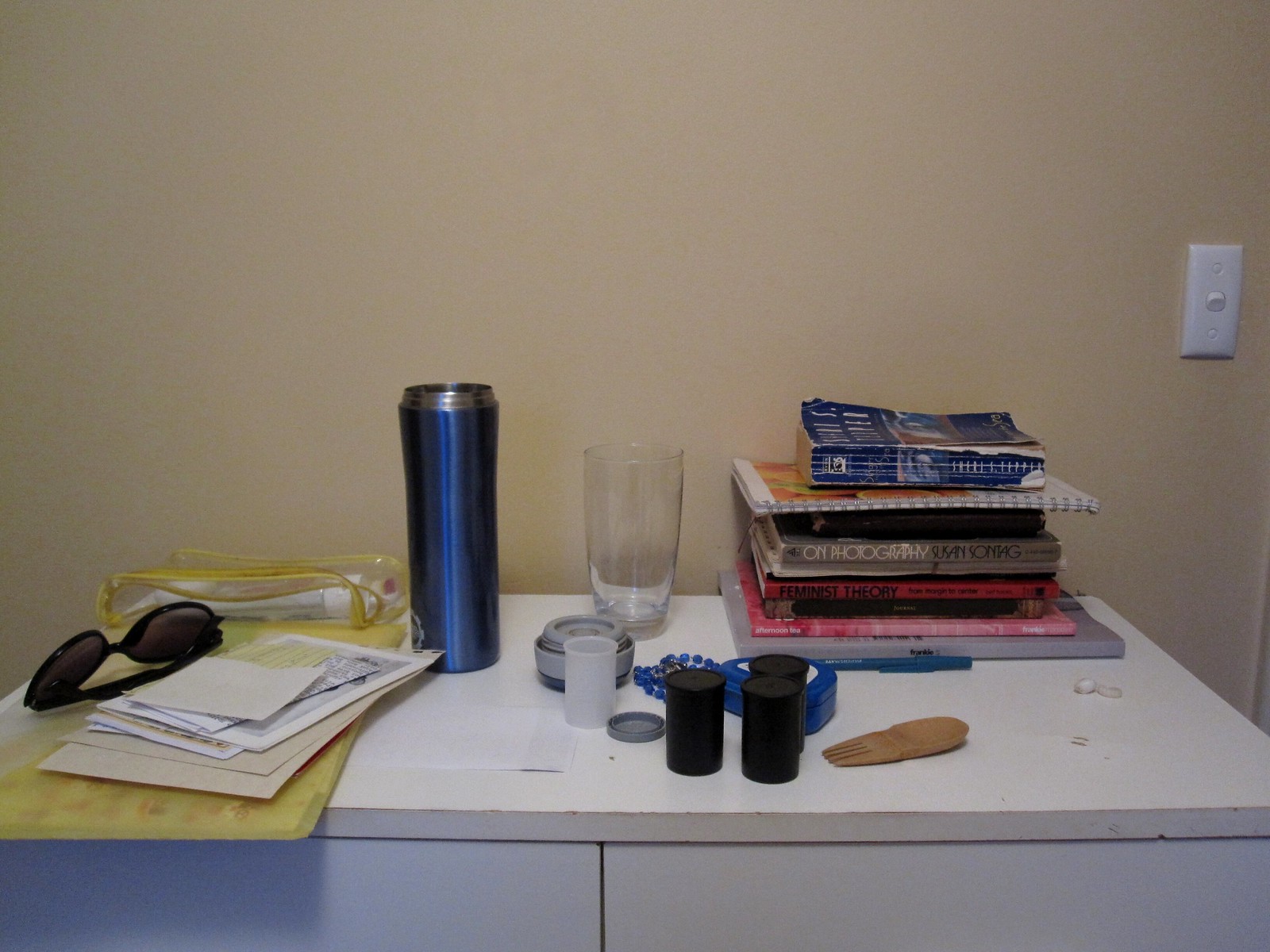This indoor photograph captures a section of a room with a brown wall featuring a white light switch in the upper right corner. At the lower part of the image, there is a white cabinet. The left side of the cabinet holds a small stack of mail, accompanied by a pair of sunglasses and a gray or clear handbag with a yellow border. Adjacent to these items is a blue water bottle or cup with a stainless steel top, the lid for which is lying next to an empty clear film canister. A gray lid is positioned nearby, along with three black film canisters. A clear drinking glass is placed on top of one of these canisters. In the upper right corner of the cabinet, a small stack of books completes the scene, contributing to the cluttered but homely setting.